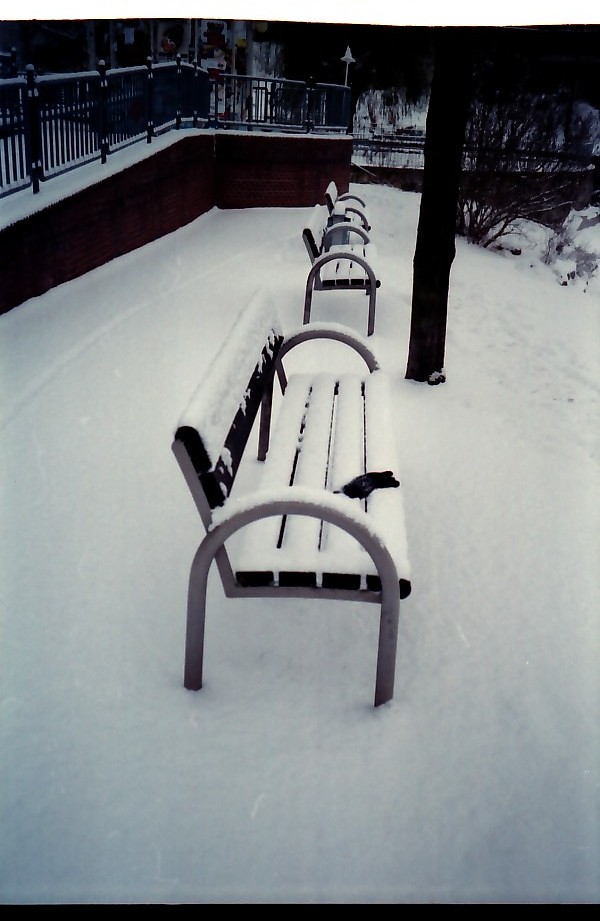The image depicts a dimly lit, wintry scene in an outdoor park-like setting. Three identical benches, lined horizontally, are covered with a thick layer of snow. A telephone pole stands between the first and second bench. Behind the benches, there is a retaining wall topped with a metal fence. Snow blankets every horizontal surface, appearing almost gray due to the flat, dim lighting. The benches are black with horizontal slats and gray, upside-down U-shaped handrails. Notably, the first bench has an object on it, possibly a glove. Trees without leaves are visible in the background, adding to the stark, monochromatic feel of the image, which also features undisturbed snow on the ground save for a possible bike trail. There is a slight incline leading up to an unseen building area, with snow drifts along the walkway.